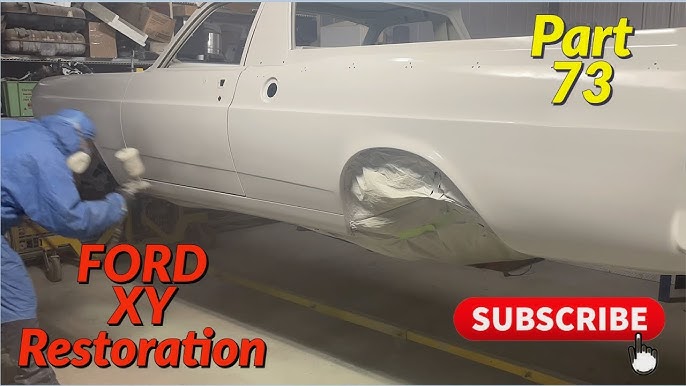The image appears to be the first page of a YouTube presentation titled "Ford XY Restoration," with this title written in red in the bottom left corner. On the bottom right corner, there's a prominent red button with white lettering that says "Subscribe," accompanied by a gray hand illustration pointing to the letter 'E'. In the upper right corner, "Part 73" is displayed in yellow letters. 

Central to the image is the side view of a vintage pickup truck, or possibly an El Camino type vehicle, which is elevated on jacks. The truck has been stripped down to its matte chrome hull, with no door handles, windows, wheels, or gas cap. Three small holes are visible along the side, likely where a top was previously attached. 

A man in a blue hazmat suit, equipped with a respirator, stands slightly bent forward on the left side of the truck, spray painting it in a cream color. He is standing on a concrete floor, and his pants are visible beneath the protective suit. In the background, metal shelving with various boxes is seen, providing a workshop-like setting.